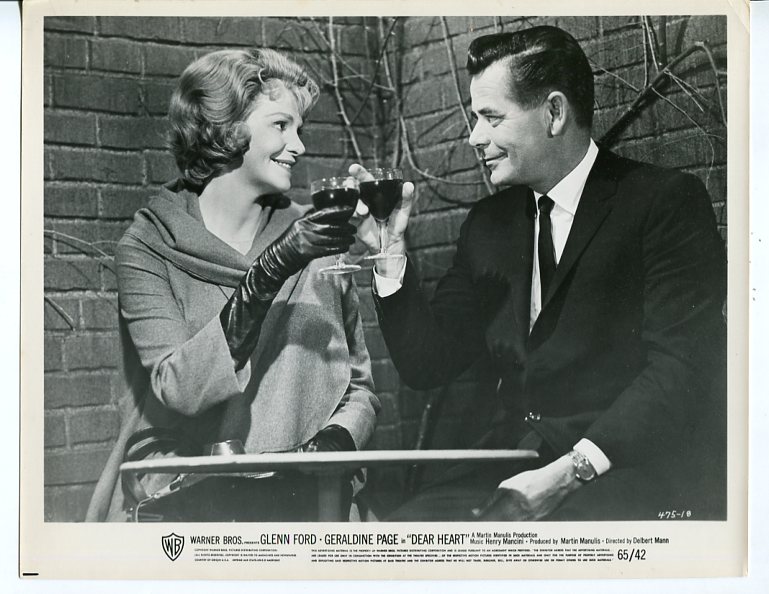This is a vintage black-and-white photograph of actors Glenn Ford and Geraldine Page, captured in what appears to be a promotional image for the movie "Dear Heart." Both actors are seated at a small table, toasting with goblets of what looks like dark wine. Ford, positioned on the right, is dressed in a formal suit and tie, with his hair slicked back and a watch visible on his left wrist. He wears a subtle smirk. Page, on the left, smiles warmly, showing a few teeth. She is elegantly attired in a long flowing dress or shawl, complemented by elbow-length dark gloves, and has short, curly hair that just reaches her neck. In the background, a brick wall adorned with bare branches is visible. At the bottom of the image, there is a classic Warner Bros shield logo, followed by the text "Warner Brothers, Glenn Ford, Geraldine Page, Dear Heart," and additional illegible writing, suggesting it functions as a vintage movie poster.